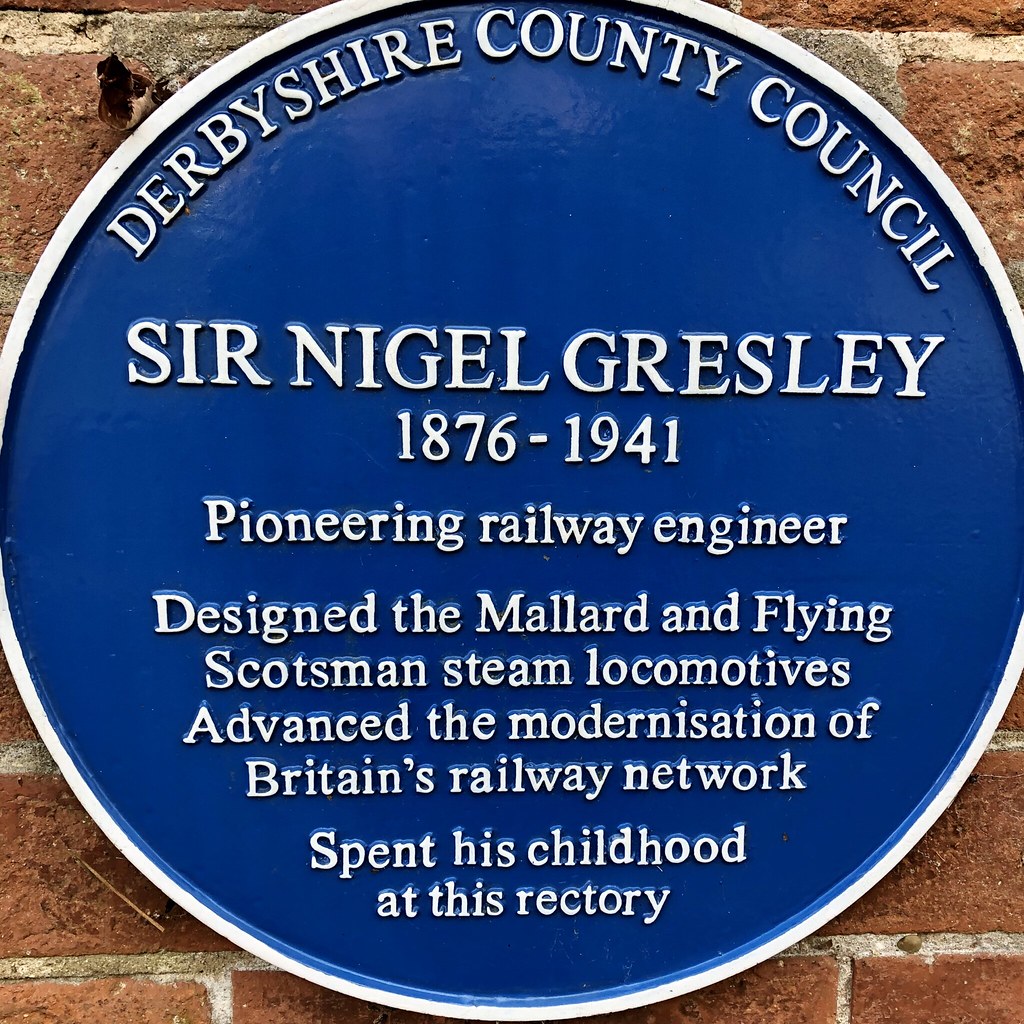The square-format, color photograph prominently features a round memorial plaque mounted on a red brick wall with white mortar. The plaque, made of metal, has a raised white border and a dark blue interior. The text at the top curves along the edge and reads "Derbyshire County Council." Below this, in all capital letters, is the name "Sir Nigel Gresley," followed by his dates, "1876-1941," presented horizontally. Beneath the dates, the plaque provides biographical details divided into three sections: Gresley is celebrated as a pioneering railway engineer, known for designing the Mallard and Flying Scotsman steam locomotives, and for advancing the modernization of Britain's railway network. The text concludes by noting that he spent his childhood at the rectory, suggesting that the brick building in the background is the rectory itself. The plaque is centrally positioned within the image and occupies most of the frame, highlighting its significance. The photographic style is a form of representational realism.